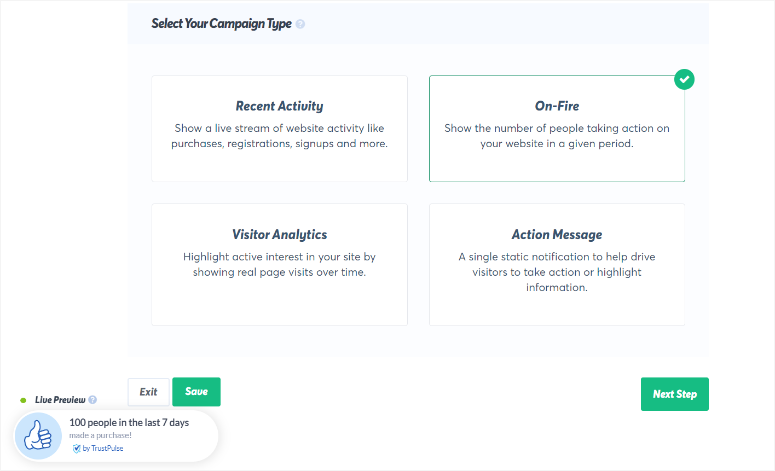This screenshot showcases a user interface for selecting a campaign type, presented against a clean, white background. At the top left, in a dark gray, slightly italicized sans serif font, it reads "Select your campaign type," accompanied by a faint question mark icon for additional information.

Below this header, several campaign descriptions are listed:
- **Recent Activity**: "Show a live stream of website activity like purchases, registrations, signups, and more."
- **Visitor Analytics**: "Highlight active interest in your site by showing real page visits over time."
- **On Fire**: "Show the number of people taking action on your website in a given period." This option features a green circle with a white checkmark icon in its top right corner, indicating selection.

Further down, the interface describes:
- **Action Message**: "A single static notification to help drive visitors to take action or highlight information."

On the bottom right corner, there is a prominent green rectangle button labeled "Next Step" in white text. 

Adjacent to this, on the bottom left, are two additional option boxes: 
- **Exit**: Displayed in a white box with black letters.
- **Save**: Presented in a green box with white letters. 

Directly beneath these options, a notification icon featuring a thumbs up in a light blue circle is visible, accompanied by a statement: "100 people in the last seven days made a purchase." Following this, there is a blue checkmark and the text "by TrustPulse."